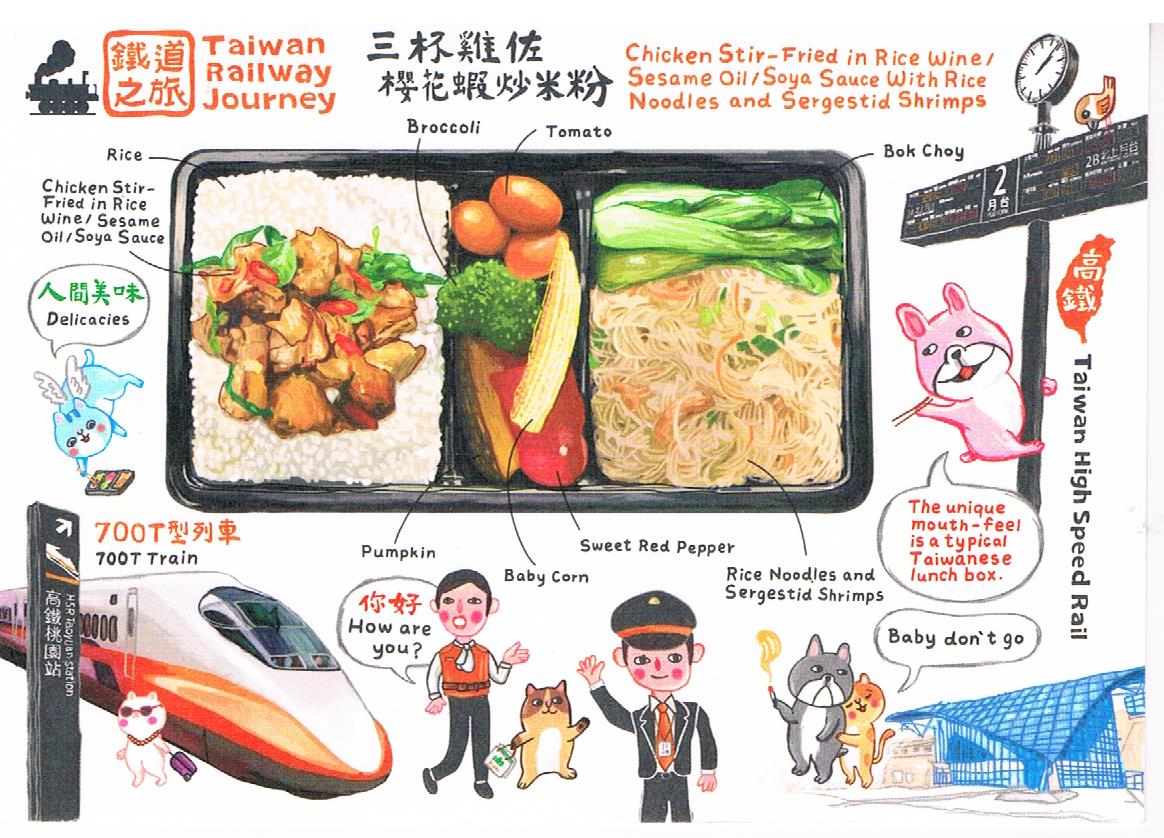This vibrant full-color ad for the Taiwan Railway Journey prominently features a black train in the upper left-hand corner, highlighted alongside Taiwanese writing and the title "Taiwan Railway Journey." The ad's background is predominantly white with various lively, cartoon-like characters surrounding the main focus, a digitally created three-compartment tray of food.

The tray is divided as follows: 
- The left section contains rice topped with chicken stir-fried in rice wine, sesame oil, and soy sauce.
- The center section includes broccoli, tomato, baby corn, pumpkin, and sweet red pepper.
- The right section features rice noodles, shrimp, and bok choy.

Black lines with labels point to each type of food, providing clear descriptions. Additional whimsical elements include a black street sign with a clock, decorated with a bird and a pink bunny rabbit/terrier holding chopsticks, and a series of cartoon figures: an orange cat hugging a gray bulldog with a speech bubble saying, "baby, don't go," a conductor greeting passengers, a cat waving goodbye, and a blue cat with wings exclaiming "delicacies" as it reaches for the lunchbox. 

Each detail collectively showcases the essence of a traditional Taiwanese lunchbox set against the backdrop of the Taiwan High-Speed Rail, making it an engaging and detailed advertisement.